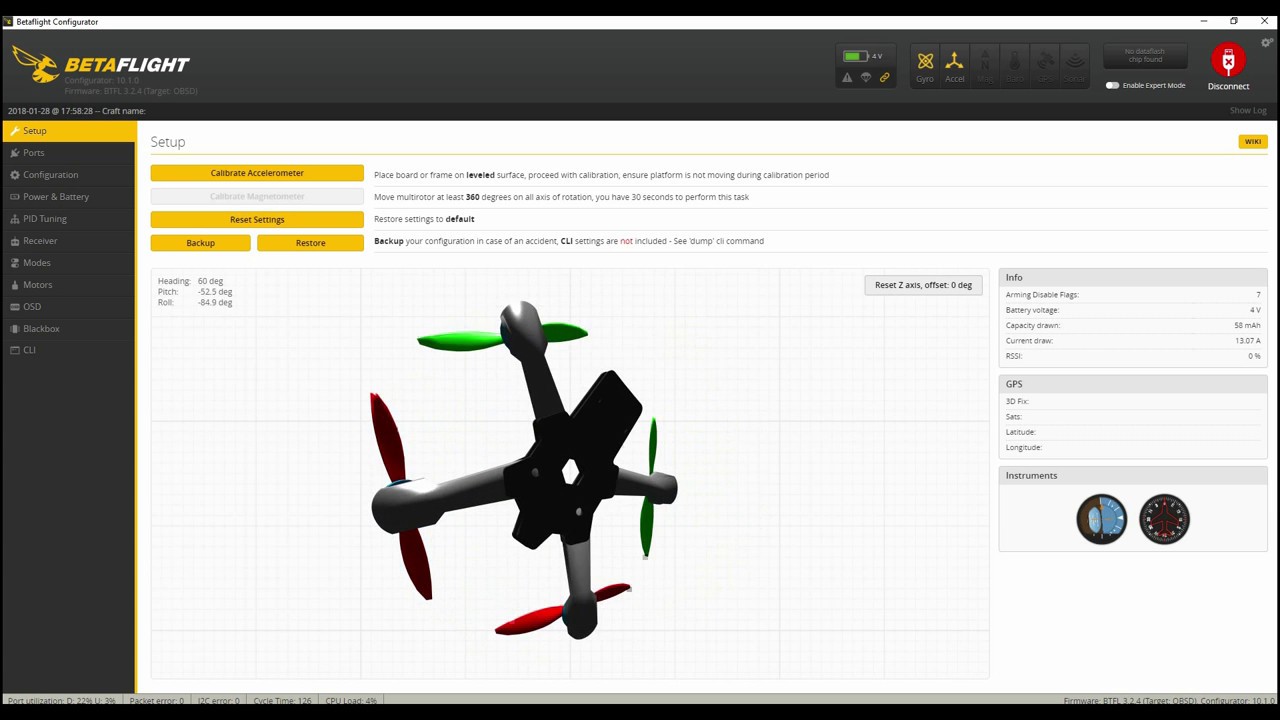The image is a detailed screenshot from the Betaflight website, a platform commonly used for drone configuration and tuning. The screenshot is expansive, making much of the text difficult to read due to its small size.

At the top, a gray bar prominently displays the Betaflight logo, wherein "Beta" is colored yellow and "flight" is in white. Accompanying the text is an icon of a bee or wasp, depicted in profile and facing right, with its stinger-curled upward.

On the extreme right of the image is a battery indicator showing an approximate 60% charge. There are various options highlighted in yellow, including what appear to be location and steering settings, while the rest of the options are grayed out. The entire interface is set against a black background.

Also visible are buttons labeled "Disable export mode" and "Disconnect," the latter represented by a red circle containing a white plug with a red X on the USB head. Below these buttons is an image of a drone, seemingly illustrating its current flight position. The drone is tilting to one side with its rear propellers displayed in green and the front propellers in red, each of its four arms equipped with a propeller.

The right side of the screenshot features multiple information panels, whereas the left side contains a vertical menu listing several options, though the small text makes them somewhat unclear. The discernible options include setup, parts, configuration, power and battery, PID tuning, receiver modes, motors, OSD (On-Screen Display), black box, and CLI (Command Line Interface).